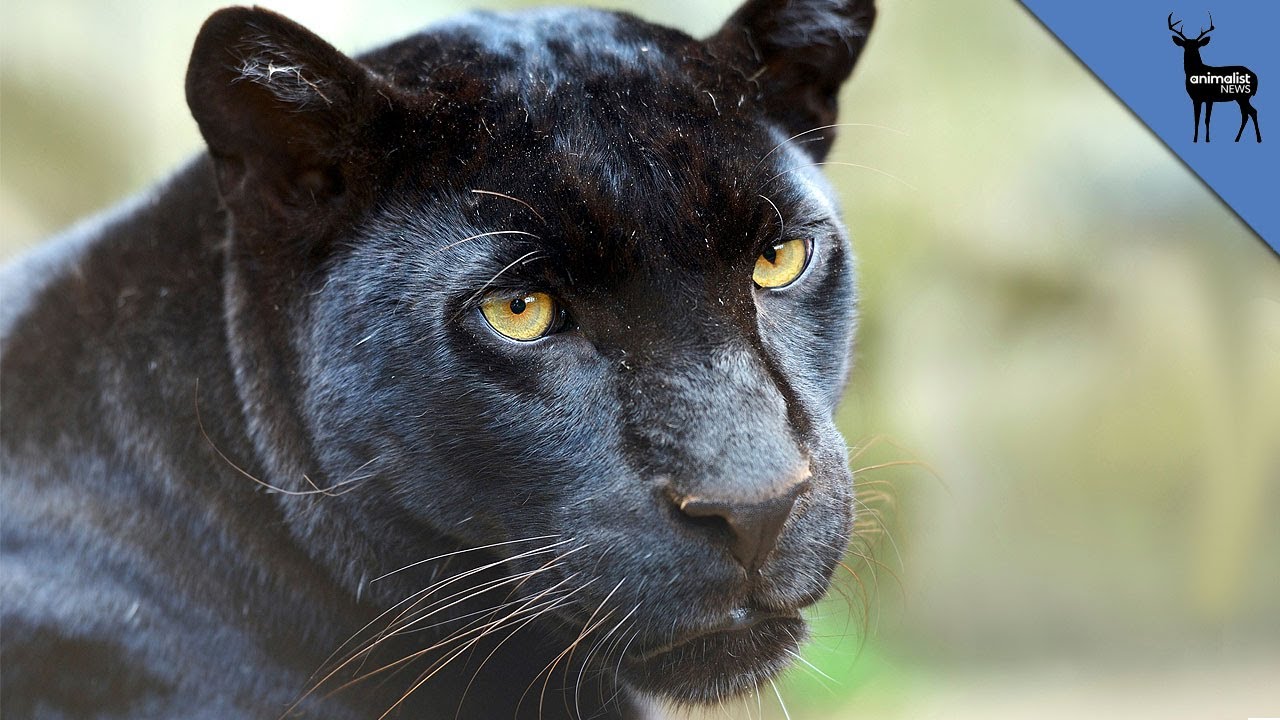The image captures an intense close-up of a sleek black panther with short, shiny black fur, staring directly at the camera with piercing golden-yellow eyes. The panther's large, prominent nose and whiskers are clearly visible, adding to its distinctive facial features. Its expression appears somewhat angry or highly focused. The background is a blurred mix of faded green, white, and possibly some berry tones, suggesting an out-of-focus forest or natural setting. In the upper right-hand corner of the image, there is a blue triangle with a logo featuring a dark brown or black deer with horns, accompanied by the text "Animalist News." The photograph has a portrait-like quality, emphasizing the panther's face, although a small part of its body is also visible.